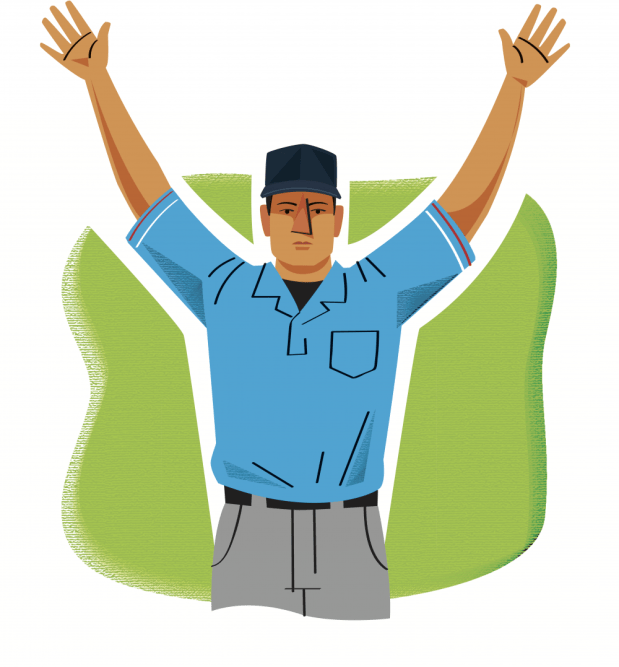This illustration depicts a computer-generated image of a male umpire or referee, drawn in a cartoon-like style. He wears a short-sleeved light blue polo shirt with a pocket and collar outlined in black, and a white and red stripe at the bottom of the sleeves. Underneath, he has on a dark shirt that is visible at the neck. His gray pants are held up by a black belt, and only the top portion of his legs is visible. The man sports a navy blue baseball cap, with dark hair peeking out from under it. His hat's visor casts a shadow over his eyes. His facial features include visible eyebrows, an angular nose, and lips. The man is depicted with his arms raised upwards, as if signaling or making a call. The background features a wavy pattern in shades of lime green and white, enhancing the focus on the umpire-like figure.